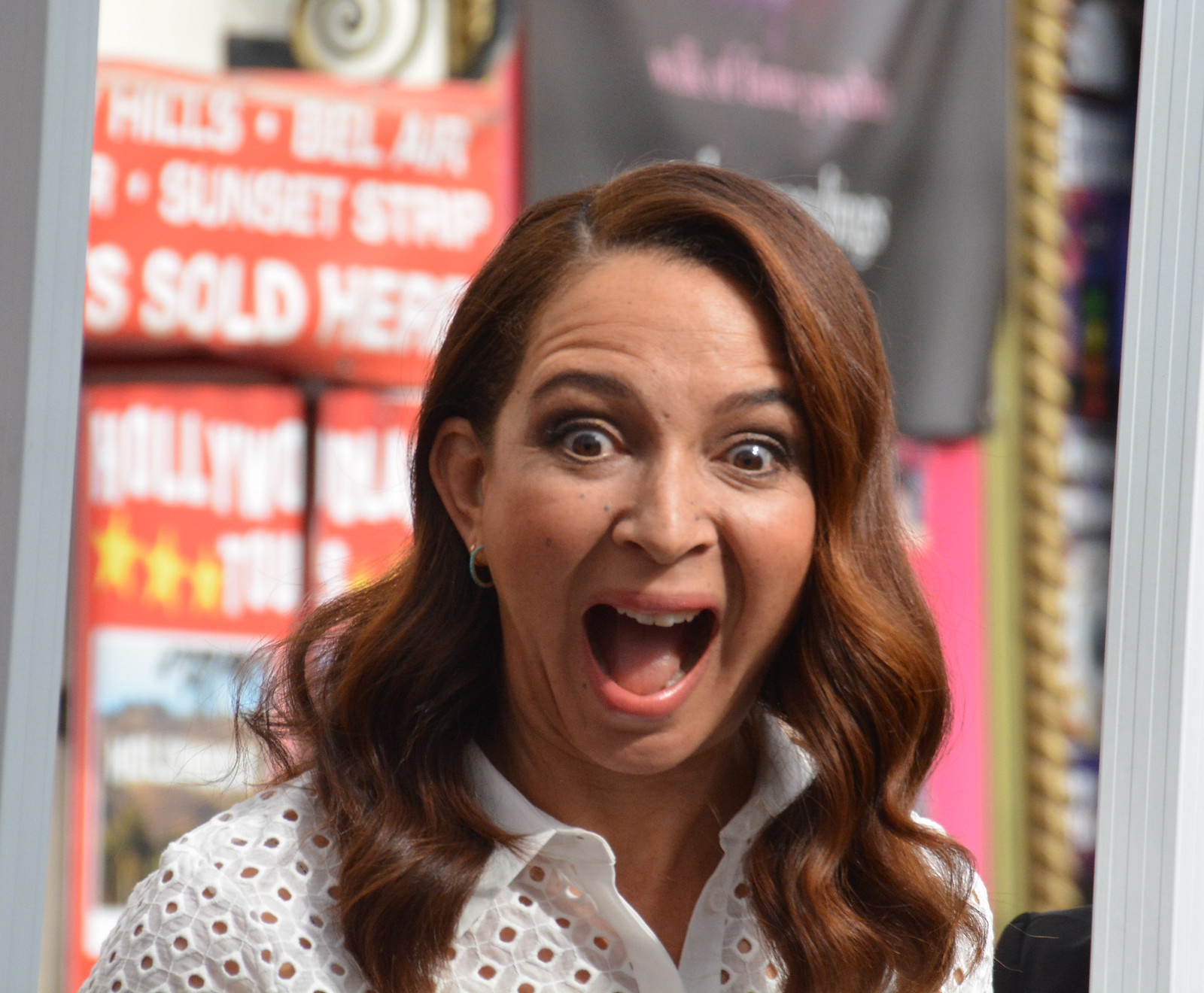In the image, a woman with long, wavy, hazelnut-colored hair cascading down to her chest is captured with a surprised and happy expression. Her mouth is wide open, her eyebrows are raised, and her brown eyes are looking slightly downward. She has brown skin and a single earring visible in her left ear, while her right ear is concealed by her hair. Notably, she also has some black moles on her cheek. She is wearing a white t-shirt adorned with an open geometric pattern, which includes triangles and possibly other shapes like squares and diamonds. The background reveals a bustling storefront area filled with various signs and banners. The signs are in red, black, and pink, and some of them read "Hills," "Sunset Strip," "Sold Here," "Hollywood," and are accented with stars. The setting appears to include elements of a wine bar, suggested by the surroundings beside her. Despite some parts being slightly out of focus, the vibrant and busy backdrop contrasts with her focused expression, adding depth to the scene.